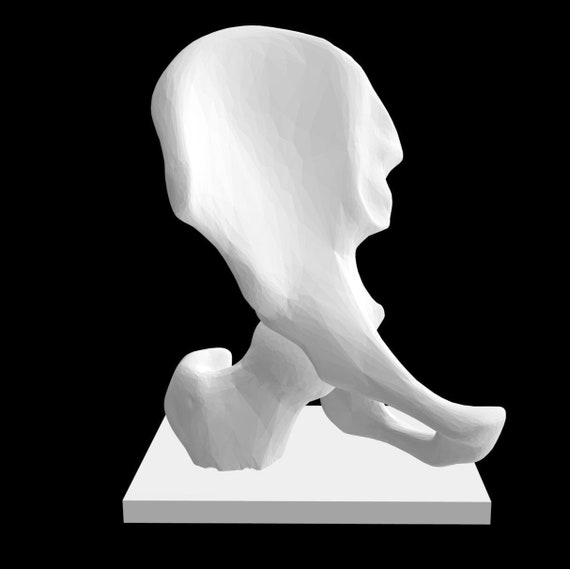The image displays a digital, white statue set against a solid black background. The statue appears to depict part of a skeletal structure, resembling the pelvis and hip bone. It is mounted on a square pedestal. The top of the figure is broad and flat, suggesting the upper region of the pelvis, while the structure extends downward, showing intricate details of the hip area. The left side of the image shows the ball and socket joint of the femur protruding from the pelvis. Two elongated, crisscrossing extensions near the bottom of the statue connect and separate, creating a small gap and adding a tripod-like appearance to the base. The entire statue, with its detailed curvature and structure, gives an impression of being made from ceramic or porcelain.